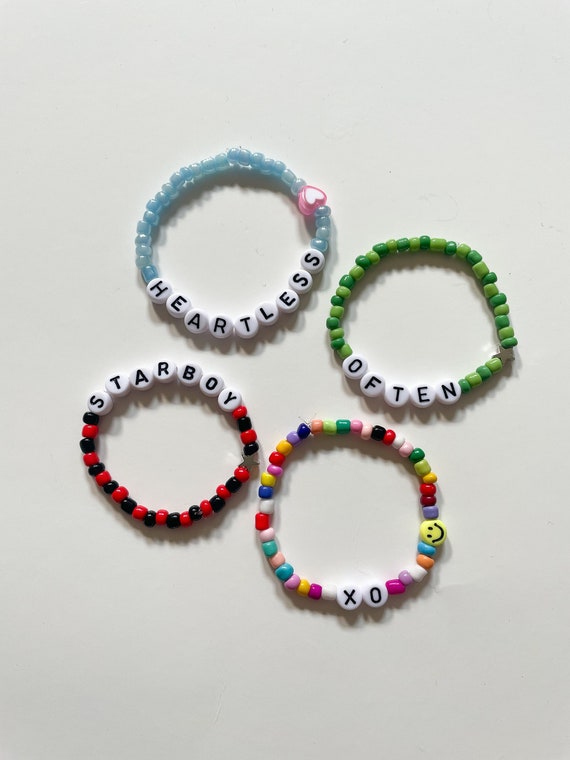This image showcases a set of four friendship bracelets arranged on a white surface, slightly off-center to the right. 

- The top-left bracelet is composed of light blue beads, featuring a white-centered heart bead and the word "heartless" spelled out in individual pieces.
- To its lower right, a bracelet alternating between lighter and darker green beads spells "often."
- Below the green bracelet is a multicolored one, exhibiting brighter hues in the top half and pastel shades in the bottom half of the circle. This bracelet includes the letters "XO" and a yellow smiley face bead on the right.
- Slightly above and to the left of the XO bracelet is a red and black beaded bracelet, with the words "Starboy" written with detailed beads. 

The bracelets are carefully arranged, each with distinct colors and unique messages, symbolizing the individuality and creativity in friendship tokens.